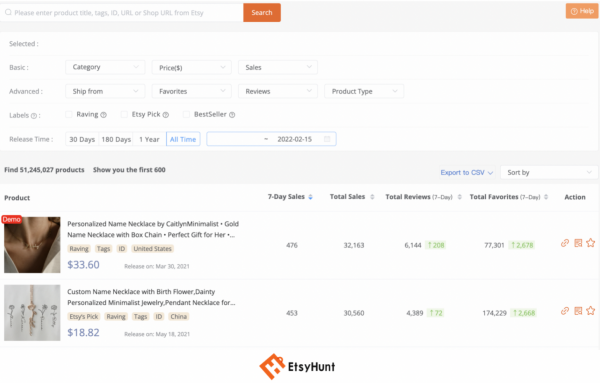**Caption for the Image:**
In the top left corner, there is an orange icon labeled "Search Help". Below, several categories are selected including "Basic", "Price", "Sells", "Advanced", "Ship From", "Favorites", "Reviews", "Prototype Labels", "Raving Etsy Picks", and "Bestseller". There is a drop-down menu for "Release Time" with options such as 30 days, 180 days, one year, and all-time. The search results indicate 151 million, 245 thousand, and 27 products, and show the first 600 results. A blue button labeled "Export to CSV" is available for data export.

The products are sorted by "Product Name". In the main section to the right, the user can view Sunday sales, total sales, total reviews, Sunday reviews, total favorites, Sunday favorites, and actions like speed red demo.

Highlighted is a popular product: a personalized name necklace by Caitlyn Minimalist, named the "Goal Name Necklace". It's marketed as an ideal gift, with a total of 60,476 sales and 32,163 units sold on a specific Sunday. The item has garnered 6,144 reviews and is favorited 7,031 times. Additionally, there's an illustration of a bird and a flower, possibly part of the necklace design, adding a touch of charm to its young, modern aesthetic.